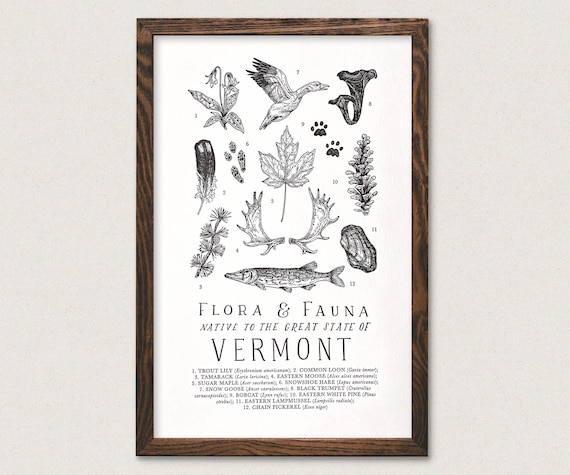This image features a rectangular framed poster with a dark wooden frame, possibly walnut, and a white background. The poster presents an array of simple black pencil illustrations reminiscent of a vintage nature textbook or Darwin's notebook. The drawings depict various wildlife and botanical elements that are native to Vermont, including a duck, a maple leaf, moose antlers, a feather with a hint of white at the bottom, an oyster or eastern lamp mussel, a flowering plant, and what appears to be an eastern white pike fish. The illustrations are clustered towards the top part of the poster.

Each illustration is numbered, and these numbers are cross-referenced with a list at the bottom of the poster, identifying the species such as the lily, loon, moose antlers, and more. Beneath the illustrations, the title reads in large, stylized text: "FLORA & FAUNA." Below the main title, in smaller italic text, it states, "native to the great state of," with "VERMONT" prominently displayed in larger font. The detailed description of each illustrated specimen and the combination of aesthetic and informative elements highlight the diverse natural heritage of Vermont.